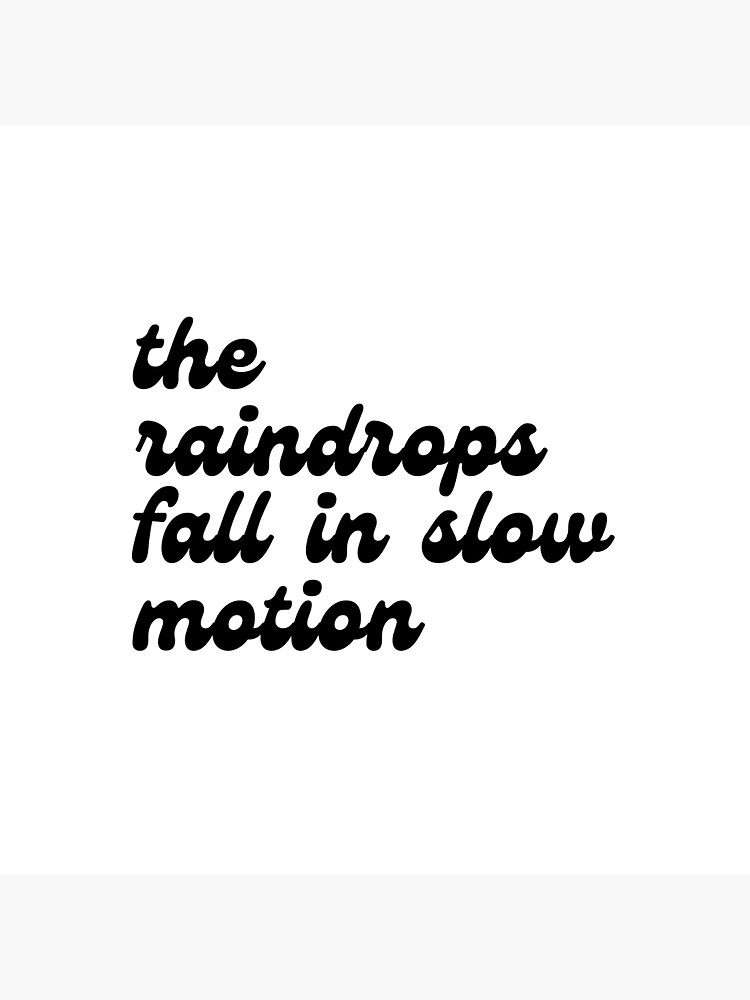The image shows a plain white background with the text "the raindrops fall in slow motion" elegantly printed in black cursive. The text is arranged in four separate lines, with "the" on the first line, "raindrops" on the second, "fall in slow" on the third, and "motion" on the fourth, all aligned to the left. The font is a beautiful cursive without any elaborate calligraphy flourishes, and all the letters are in lowercase. Just above the bottom edge of the image is a slightly darker, grayish rectangle running horizontally across the width, adding a subtle visual element. The fine detailing suggests the use of a fountain pen, enhancing the artistic presentation of the simple yet evocative phrase.